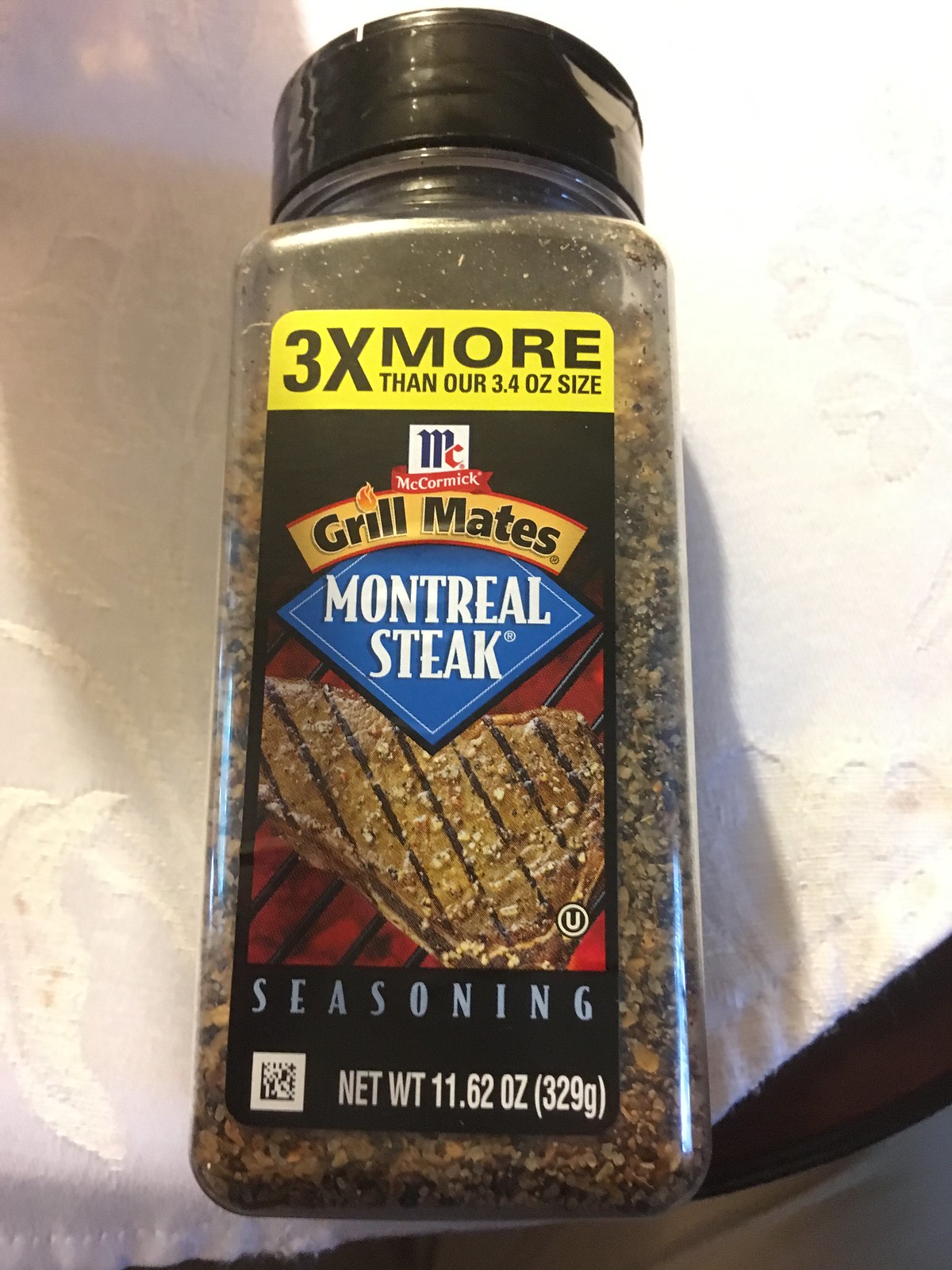The image depicts a plastic bottle of McCormick Grill Mates Montreal Steak Seasoning, which is approximately 50% taller than it is wide. The bottle, which is laying on its back with the label facing upward, is rectangular and slightly tapered at the top. It features a black plastic screw cap, likely the kind that allows for flipping between sprinkling holes and an open pour side. The label spans the entire front of the bottle. It has a prominent yellow banner at the top that reads "3.3 times more than our 3.4 ounce size" in black text. Beneath this, the "McCormick" label appears, followed by an arched gold-colored banner displaying "Grill Mates" in black letters and a blue diamond-shaped area with "Montreal Steak" in white letters. Below this section, there is an image of a steak with grill marks. The bottle contains 11.62 ounces of seasoning and appears to be about 80% full. The background is a whitish-gold dish towel or tablecloth with an area on the right side washed out by light, possibly from a room light or camera flash. The scene shows shadows cast from the upper left to the lower right side of the towel.